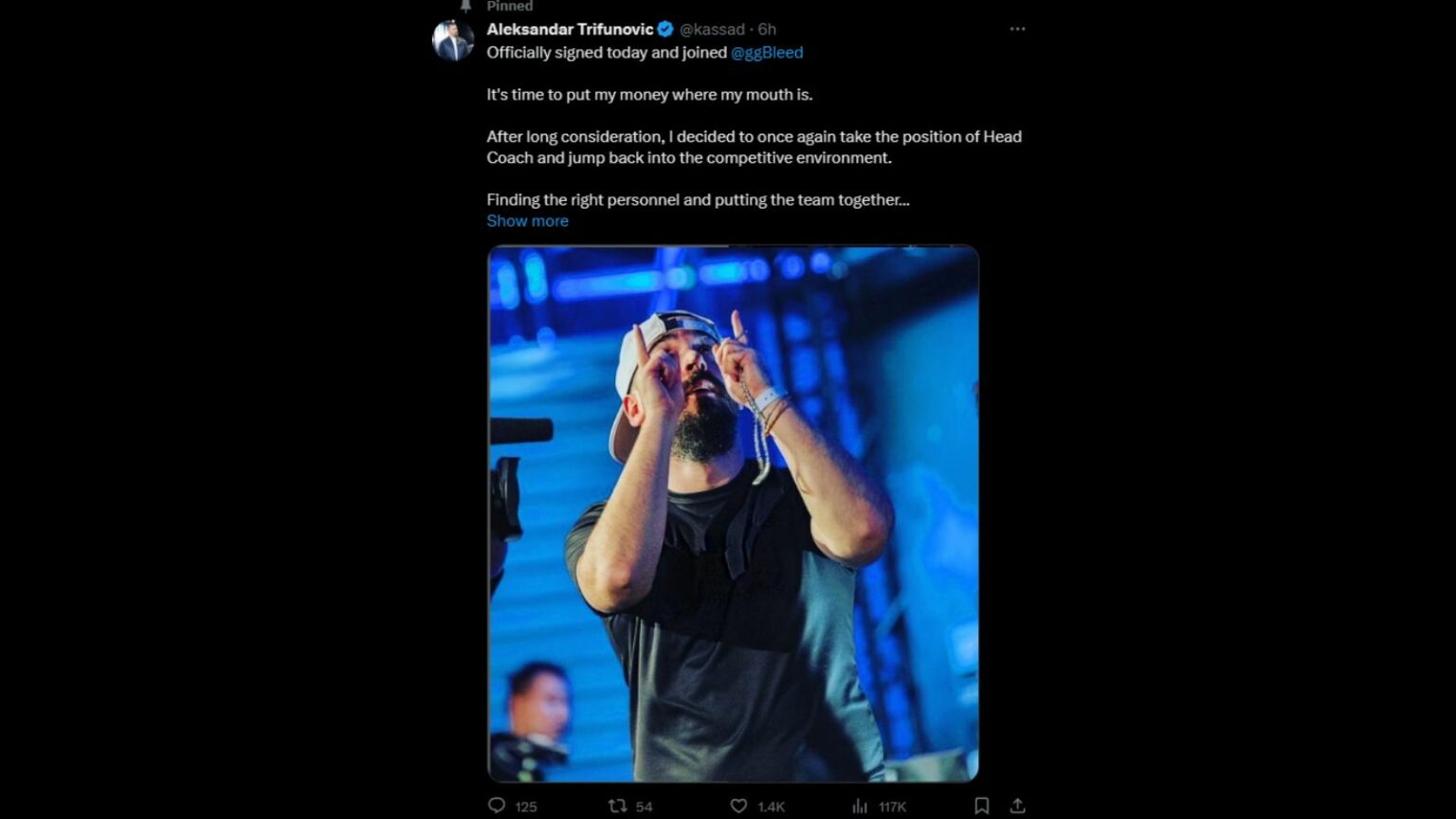**Caption:**

In a recent Twitter post by Alexander Trifunovic (@Kasad), shared six hours ago, a noteworthy announcement was made alongside a photograph that captures the moment vividly. The post has a sleek black background, highlighting the image and text. It features a small circular profile picture of Trifunovic, a man donning a blue jacket, with a notification bell icon and a pinned tag above it. 

In the attached image, Alexander Trifunovic, identifiable by his white backward baseball cap and scruffy black beard, stands against a metal-framed blue wall. He wears a gray shirt and a wristwatch along with other wristbands on his left wrist. With both arms extended and fingers pointing upwards, he seems to be celebrating or making a strong statement. A hint of a blurry figure and some camera equipment can be seen on the left, indicating a bustling environment. 

The post reads: "He was officially signed today and joined at GG Bleed. It's time to put my money where my mouth is. After long consideration, I decided to once again take the position of head coach and jump back into the competitive environment. Finding the right personnel and putting the team together…” with a continuation hinted by "show more."

Though it’s not explicitly mentioned in the post what sport or game Trifunovic will be coaching, the update indicates his return to a head coaching role, emphasizing his enthusiasm and readiness to build a team and face new challenges.